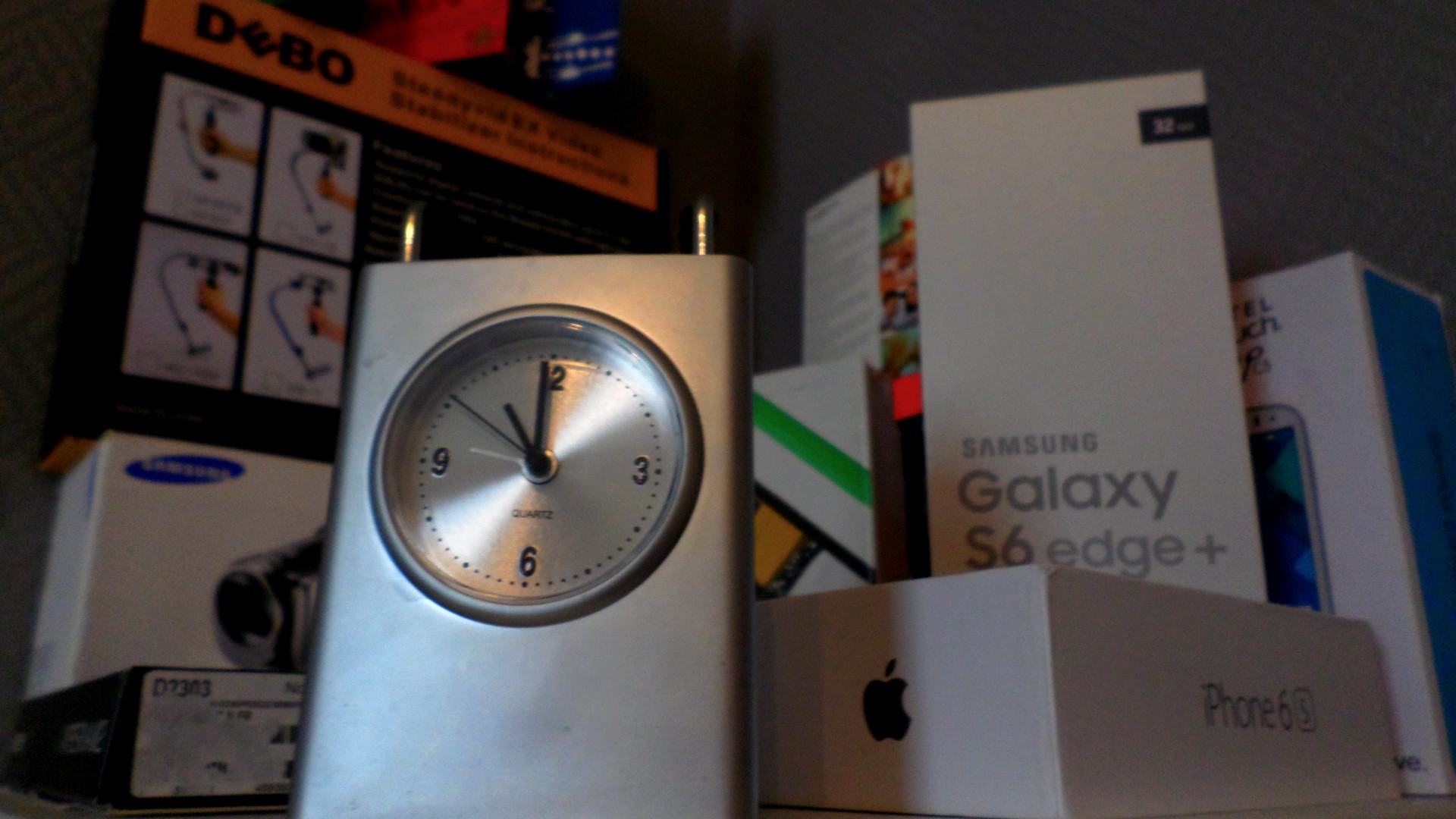The image showcases a collection of technological devices alongside their respective packaging. Prominently in the foreground is a sleek, silver rectangular case featuring a classic analog clock with a round silver face. The clock displays the numbers 3, 6, 9, and 12, with the hour and minute hands in black and a thinner black second hand. In the background, a black-and-green box labeled "Debo" in capital letters can be partially seen. To the left, a white box for a Samsung camcorder is visible, while in the bottom right corner, a white box with the Apple logo and "iPhone 6S" can be identified. Additionally, there is a white box that reads "32GB Samsung Galaxy S6 Edge Plus," completing the array of tech items and their packaging.